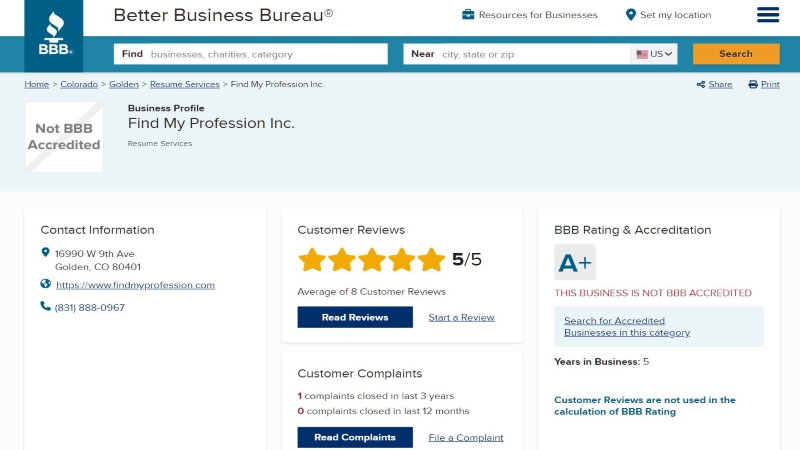This web page belongs to the Better Business Bureau (BBB). The BBB logo, located in the top left corner, is a blue rectangle featuring three capitalized letters "BBB" in white, stacked vertically, with a stylized image of a flame burning on a plate above them. At the top of the website, there are two search bars: the first prompts users to search for "Businesses, Charities, or Categories," and the second prompts users to search "Near," asking for a city, state, or zip code. A drop-down menu next to the second search bar allows users to select their country, with "US" being the default option. An orange-colored button labeled "Search" is positioned at the end of the input fields.

Below the search section is detailed information about a business profile, including contact information and customer reviews. The business currently has a perfect rating of 5 out of 5 stars, based on eight customer reviews. Additionally, the BBB rating and accreditation information is prominently displayed, with this particular business holding an A+ rating.